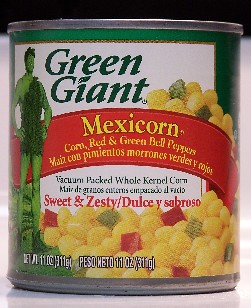This image features an 11-ounce can of Green Giant Mexicorn, prominently displayed against a plain white surface with a black background. The can has a green label with a white square on the front, and a bright red banner across the middle. The banner reads "Mexicorn" in large yellow letters, followed by a description: "corn, red and green bell peppers," with the same information written in Spanish below. The lower portion of the label showcases an appetizing image of golden-yellow vacuum-packed whole kernel corn mixed with vivid red and green bell pepper specks, described as "sweet and zesty." 

Standing on the left side of the can is the iconic Green Giant figure, depicted with green skin and hair, wearing a leafy tunic, green tights, and leaf-adorned shoes. His hands rest confidently on his hips. The can has a silver rim, completing its overall appearance.